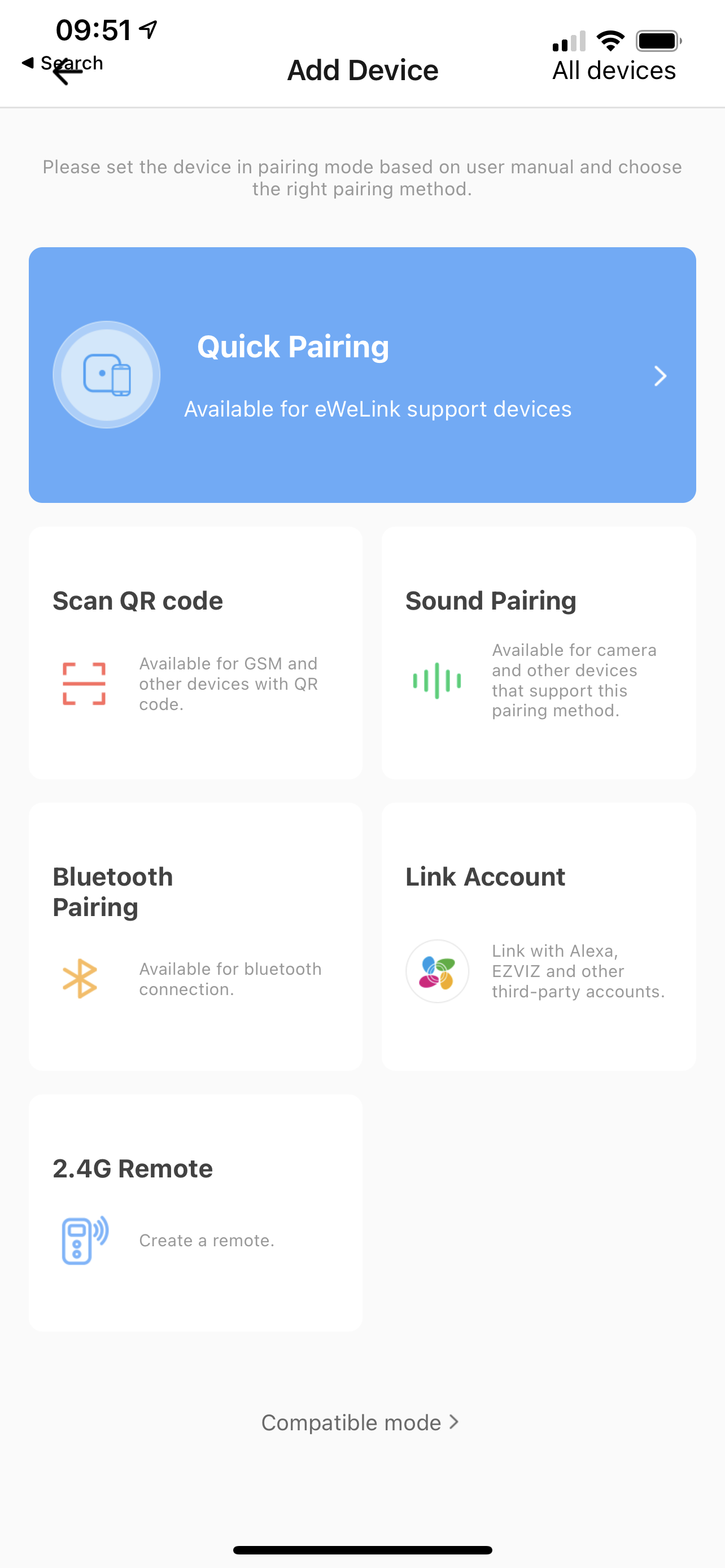This is a screenshot of a device screen, possibly a smartphone or computer. The time displayed at the top left corner is 09:51 in black text. Directly beneath the time, "Add Device" is written in black text. Moving to the right, there is a full black battery icon indicating a full charge. Below this, "All Devices" is written in black text.

The central portion of the screen features a blue rectangle with white text that reads, "Quick pairing available for e-wheeling support devices." Below this, in black letters, it says, "Scan QR code." Further to the right, "Sound Pairing" is written in black text, accompanied by several green lines underneath it.

Beneath these sections, "Bluetooth Pairing," also in black text, is displayed with an orange Bluetooth icon situated below it. Below this, the screen reads, "Link Account" in black text followed by "Link with Alexa" in black and gray text.

In response to an input or command, the text "Sorry, I don't have an answer for that" is displayed, indicating the system did not understand a previous query or command.

Near the bottom of the screen, "2.4G Remote" is written in black text, followed by "You can create a remote," also in black text. This description is accompanied by a blue icon of a phone. At the very bottom of the screen, there is a solid black line, which might indicate a separator or the edge of the screen interface.